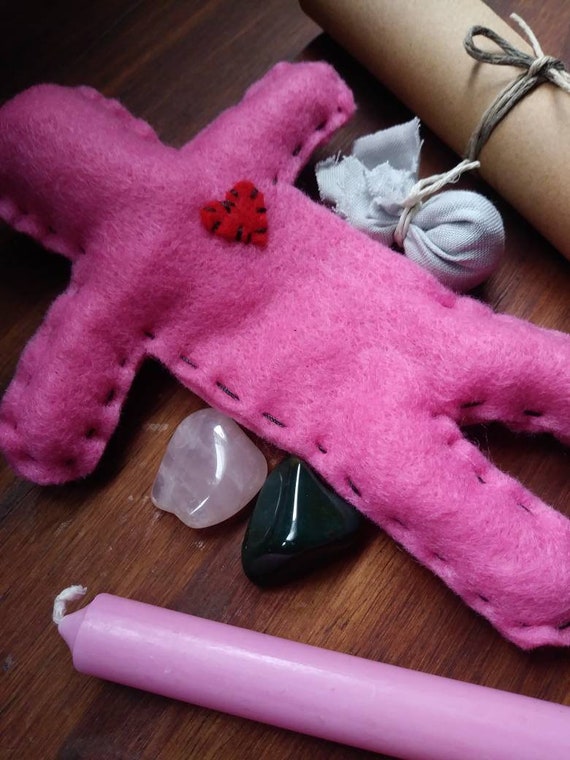This close-up vertical photograph showcases a carefully arranged assortment of items on a reddish-brown wooden table. Dominating the center of the image is a simple, bright pink felt doll designed in the form of a stickman. This doll, stitched in black around its edges, features a small red felt heart secured to the right side of its chest with black stitches, possibly evoking a handmade or voodoo-style aesthetic.

Beneath the doll, near its sides, rest two polished stones: a shiny, curved-edge pink stone to the left and a solid, shiny black stone to the right. At the very bottom of the frame, a pink candle lies at an angle with its white wick pointing to the left, adding a subtle touch of color contrast against the wooden background.

Above the doll, a small white fabric bag tied tightly with a piece of string sits to the right, suggesting a sense of mystery or hidden content. Further up, mostly cut off by the top and top-right edges of the frame, a rolled-up piece of brown paper tied with brown string is visible, resembling a coiled piece of grocery bag material or card stock.

Together, these elements form a visually intriguing composition, combining textures and colors in a tidy but mysterious arrangement.